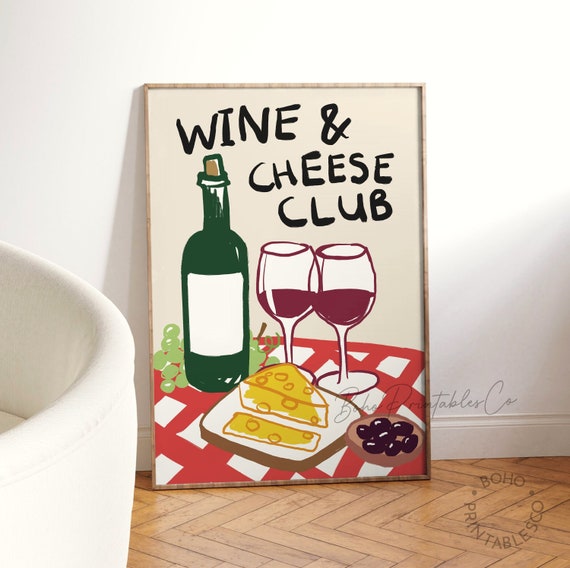The image features a painting as its primary focus, with the painting propped up against a white wall. The foreground showcases a hardwood floor with a distinct spiral back-and-forth design. To the left of the image, the edge of a white sofa or chair can be partially seen. Centrally positioned, the painting reads "Wine and Cheese Club" in black text against a white background. Situated in the bottom part of the artwork is a checkered table bearing two wine glasses filled with wine, a green wine bottle with a cork still in it, a plate of grapes, and two slices of cheese on a small platter. Additionally, there are some olives depicted on the table. The entire scene is detailed, creating an inviting and cozy atmosphere.